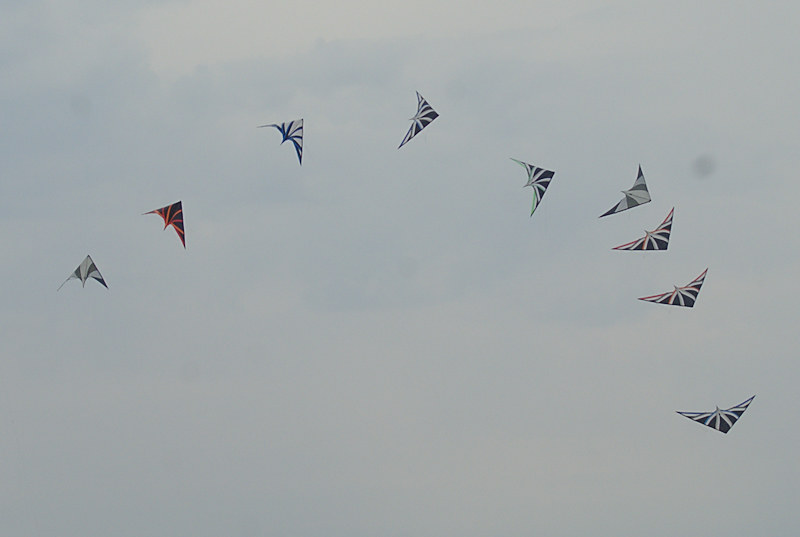This color photograph depicts a dynamic scene of nine paragliders in flight against a light blue sky, adorned with thin white clouds. The paragliders form an upward-arching, partial circle, giving the appearance of a fan or a sequence captured mid-motion. Each paraglider exhibits a uniform triangular shape with distinct, striped patterns. The primary colors of the paragliders range from white, navy blue, red, turquoise blue, gray, and combinations with black. The scene suggests a possible time-lapse effect, starting from the top left to the bottom right, adding a layered visual depth. Despite the cloudy atmosphere, the vivid colors of the paragliders create a striking contrast against the muted sky, capturing the essence of a cloudy but visually captivating day.